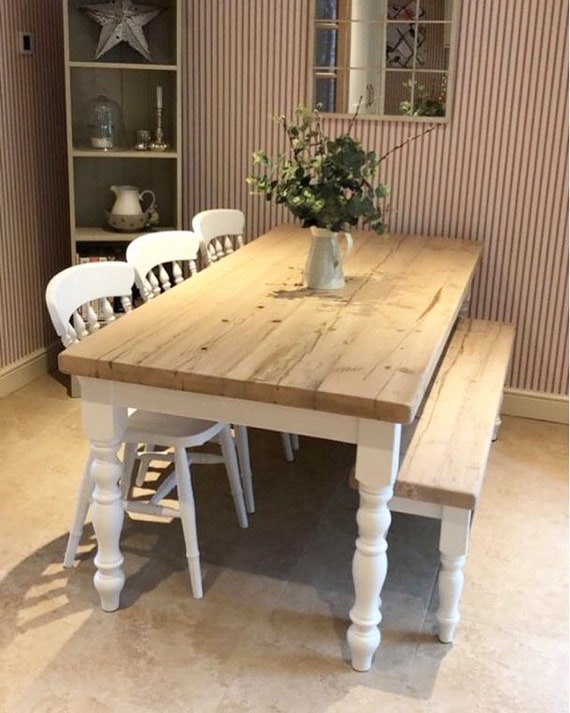The photograph captures a charming and rustic farmhouse-style dining or kitchen area. The centerpiece is a table with a light tan wooden slat tabletop and white wooden legs. On the right side of the table is a matching wooden bench with white legs, partially tucked under the table. Across from the bench, on the left side of the table, are three white wooden chairs. The table features a white milk pitcher with green sprigs and plants arranged in the center. Behind the table, the wall is adorned with vertical red and white striped wallpaper. A window or perhaps a mirror with panes is positioned above the table on this wall. The flooring is a peach-tan colored stone or marble that complements the room's rustic aesthetic. In the corner to the left, there is a light beige bookshelf holding various decorations, including a star, a glass clock, a candle, and a water pitcher, adding to the home's cozy charm.